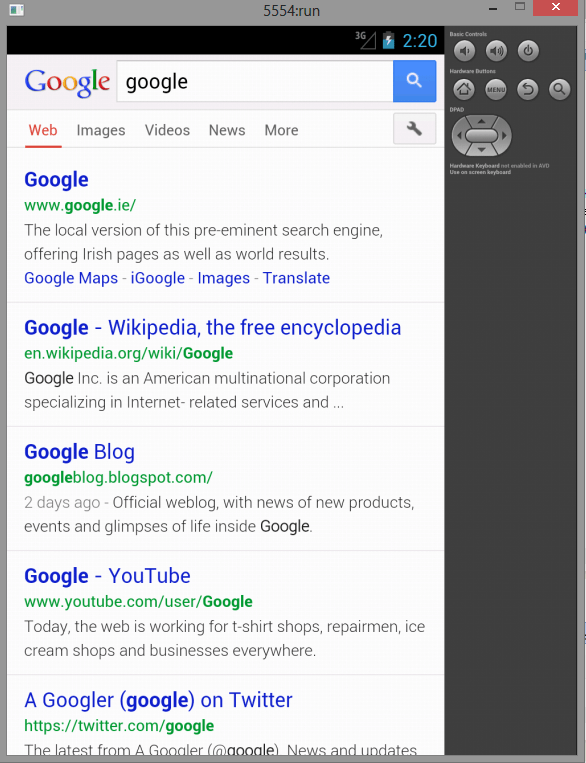This image depicts a screenshot bordered in gray against a black background. The upper gray header displays "5554 run." In the upper right corner, there is a white "X" inside a red square. Below this, on a white background, the Google logo is shown with its iconic colors, accompanied by a search box containing the word "Google" in black text. A white magnifying glass icon is present within a blue search button.

Underneath the search bar, "web" is highlighted on the left side in red text and underlined. To the right of "web," the options "images," "videos," "news," and "more" are displayed. An icon of a wrench inside a gray box is positioned further to the right.

Below this navigation bar, the text "Google" appears in blue, followed by the URL "www.google.ie" in green, indicating the regional version of the search engine tailored for Ireland, offering both local and global search results. Below the URL, options such as "Google Maps," "iGoogle," "images," and "translate" are listed.

At the bottom of the image, there is a reference to Google's Twitter account, stating: "A Googler Google on Twitter https://twitter.com/Google."